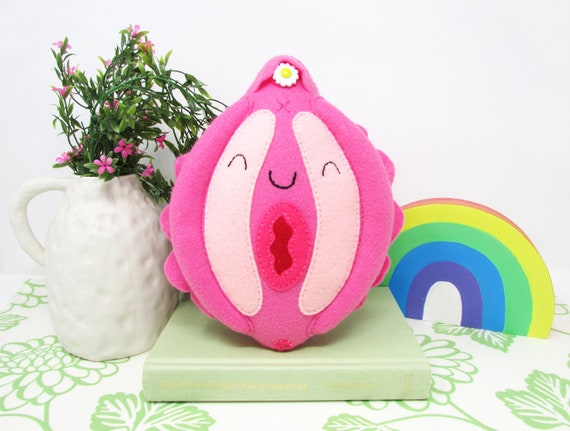The image showcases a collection of items arranged on a white tablecloth adorned with green floral designs. Central to the composition is a pink plush toy resembling a female organ with a smiley face and a flower atop it, resting on a green book with white text on the spine. To the left of the plush toy is a white ceramic jug featuring a handle, filled with green stems and tiny red sunflowers that droop slightly. On the right is a medium-sized, colorful 3D wooden block figure of a rainbow, displaying the typical hues of red, yellow, green, blue, and purple. The overall background of the photograph is white.